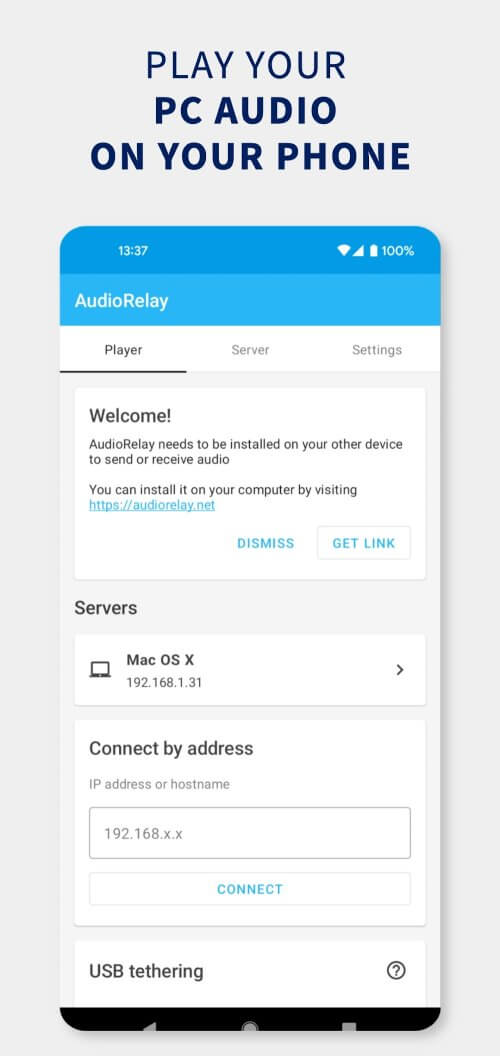The image features a prominently displayed header that reads "Play your PC audio on your phone." Below, a smartphone screen is depicted with a blue banner at the top containing the text "Audio Relay." The interface shows different tabs labeled "Player," "Server," and "Settings," with "Player" being highlighted by a black underline and displaying a welcome message.

The message explains that "Audio Relay" needs to be installed on the other device to send or receive audio. It provides a link to download the software from the website https://audiorelay.net. Adjacent to the link are two blue buttons labeled "Dismiss" and "Get Link."

Under the "Server" tab, it lists "macOS X" and an IP address, "192.168.1.31." It offers connection options via address, IP address, or hostname, with a pre-filled box showing "192.168.x.x." Next to the box, there is a blue "Connect" button. The section also includes a "USB tethering?" question mark prompt.

The bottom of the screen features a black border with gray buttons and a black arrow.